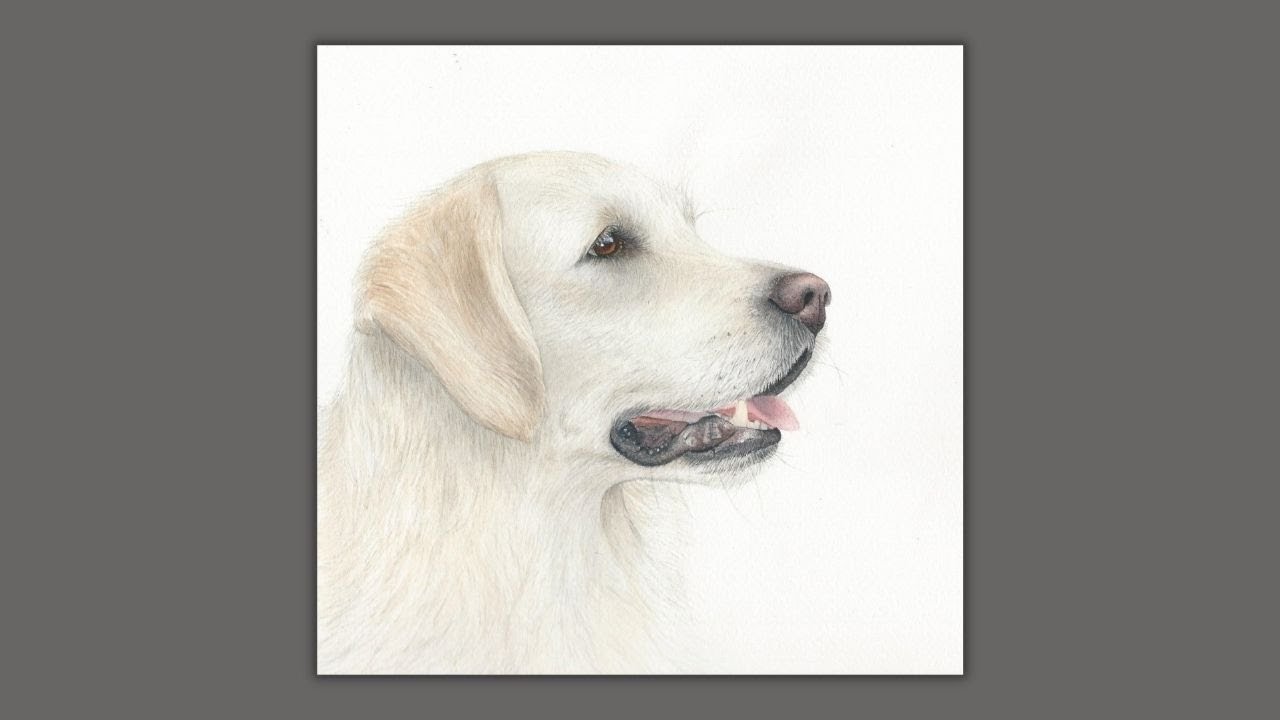The image depicts a detailed drawing of a young English Golden Retriever, characterized by its white fur with hints of cream and brown, adding depth and texture. The dog's ears, slightly darker with more brown, hang down gently, and its expressive brown eyes look to the right in a side profile, giving an impression of curiosity or alertness. The retriever's mouth is open slightly, revealing a pink tongue and a glimpse of a tooth, with black lips contrasting against its light fur. The image is set against a white background, providing a clear contrast to the dog's light blonde coat, and this white square is framed by a gray rectangle, possibly indicating it is laid on a gray countertop or surface. The meticulous use of colored pencils is evident in the nuanced shading and detail captured in the fur and facial features.